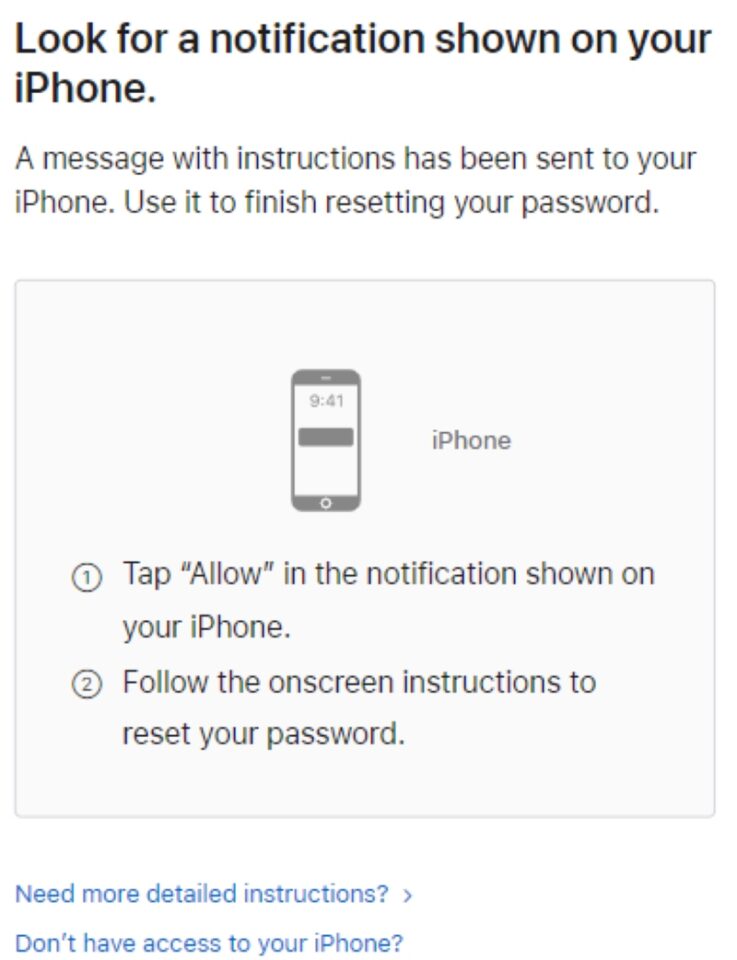**Descriptive Caption:**

The image provides a step-by-step guide for resetting the password on an iPhone. It features prominently an instructional message in black text directing users to look for a notification on their iPhone that contains a message with further instructions on completing the password reset process. This method is applicable only to iPhone users who have forgotten their password.

Within the image, there is a gray square that contains a visual representation of an iPhone, clearly labeled with the word "iPhone" next to it. Below this, two steps are detailed within the same gray square:
1. Step One (circled in the image): "Tap allow in the notification shown on your iPhone."
2. Step Two (circled in the image): "Follow the on-screen instructions to reset your password."

Beneath this instructional gray square, the image includes a section of blue text stating, "Need more detailed instructions?" accompanied by a clickable arrow. Following this, a black text line asks the question, "Don't have access to your iPhone?" without an accompanying arrow. This segment suggests seeking additional help or details if access to the iPhone is an issue.

This instructional guide is intended for iPhone users exclusively, offering a clear and detailed process for resetting a forgotten password using on-screen prompts and notifications.